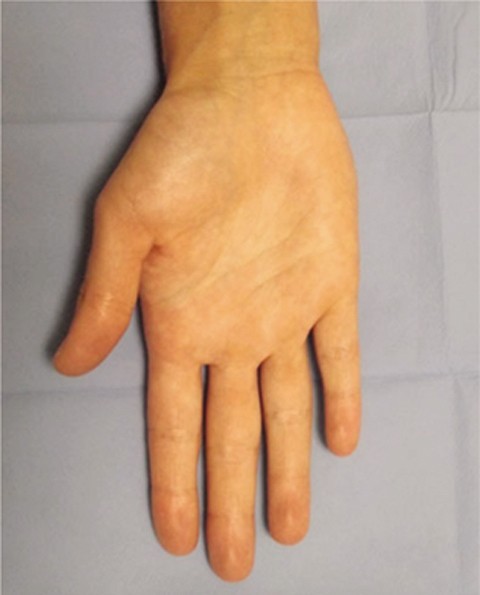The photograph features a close-up of a right hand belonging to a person with light-toned skin. The hand is lying flat with the palm facing upwards and the fingers, including the thumb and wrist, pointed towards the bottom of the image. The background is a sterile-looking blue cloth, possibly resembling medical fabric. The hand's fingers are mostly together with a slight spread, emphasizing the length of the middle finger. The detailed, almost shiny skin texture, includes visible lines and the subtle visibility of space between the fingers. The setting gives the impression of a clinical or clean environment, with no other objects present in the frame.